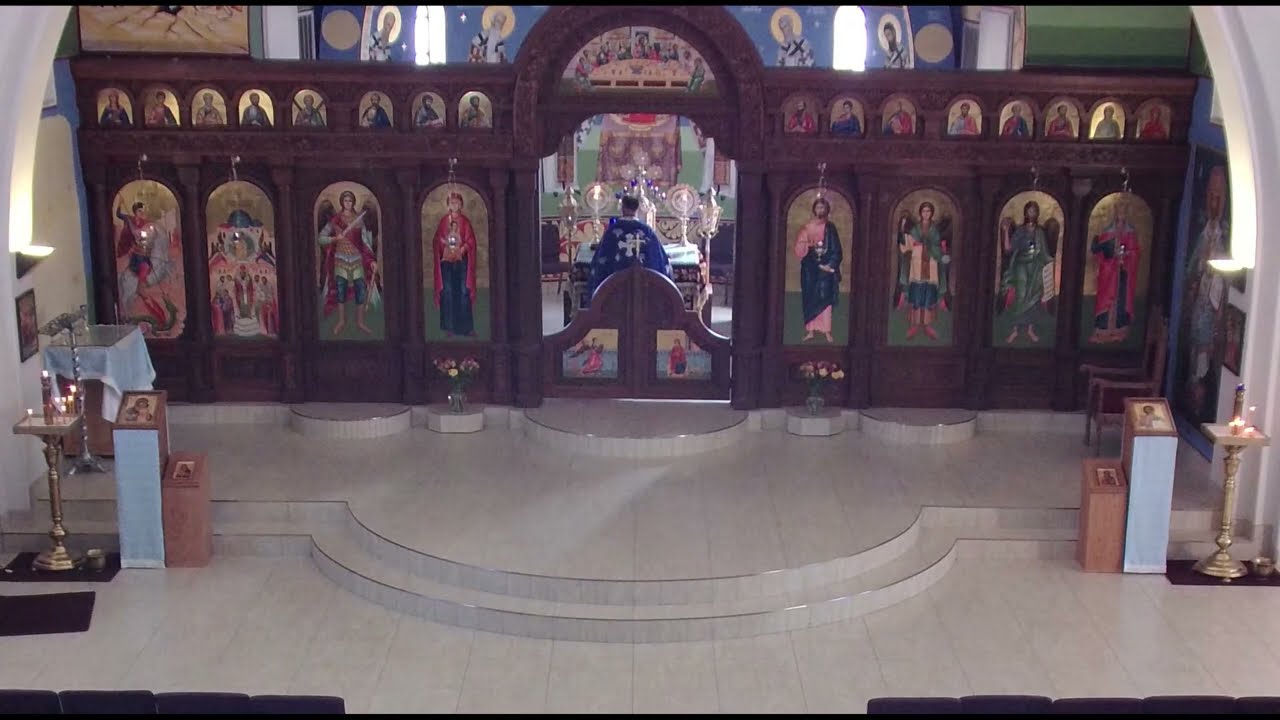The image depicts the interior of an ornate church, featuring a prominent raised white stone platform accessible by a few steps. At the center of the platform stands an archway with a person in a blue robe, adorned with a cross, facing away from the viewer. This individual is positioned in front of a large altar, decorated with gold candles and various other gold ornaments. The backdrop of the altar is an intricately carved brown wall, showcasing vibrant, pre-Renaissance-style portraits of religious figures and angels. Above the central space, there are numerous smaller, colorful paintings. The floor appears tiled and new, contrasting with the potentially ancient or expertly reproduced artwork on the walls. Flanking the platform are smaller side tables and raised plaques on pedestals, accompanied by candles. Additional statues and artistic designs adorn the background, enhancing the sacred ambiance of the setting. The entire scene is bathed in rich hues of white, brown, gold, light blue, red, green, and yellow, further emphasizing the church's historical and artistic significance.